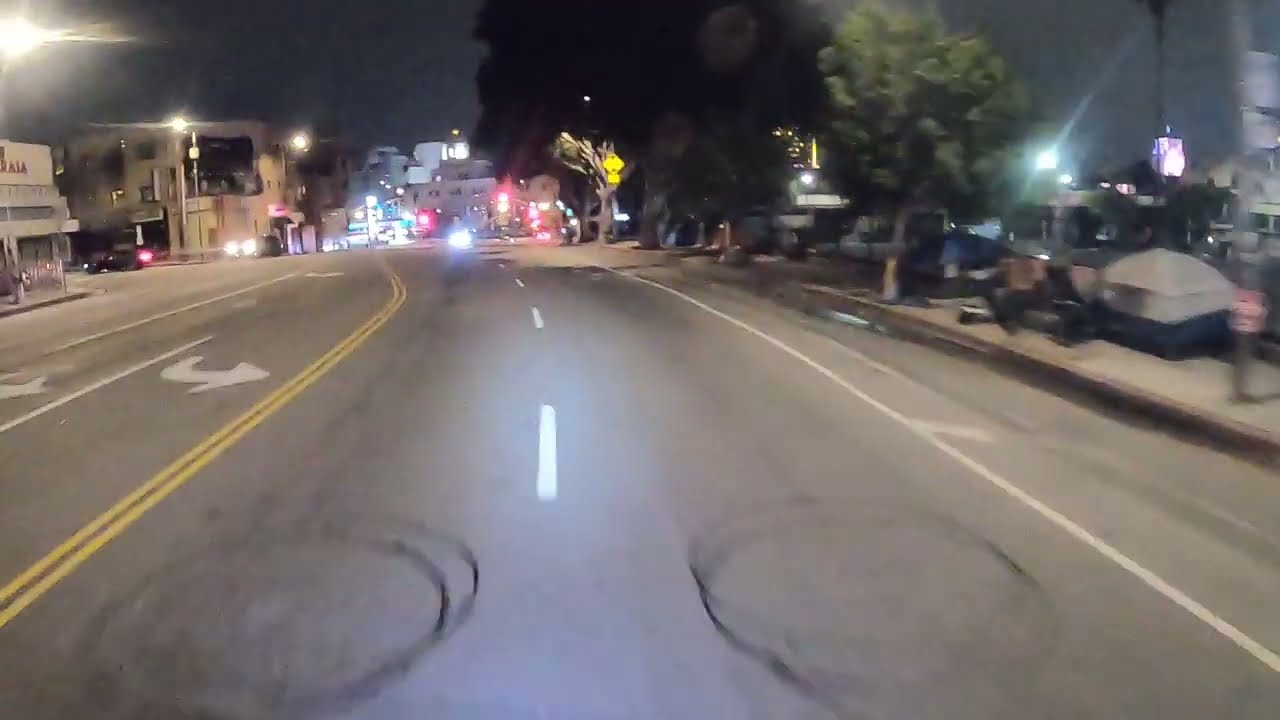The image captures a bustling downtown city street at night, illuminated by streetlights lining both sides of the road. The asphalt street features distinct white pavement markers, lane dividers, arrows, and a prominent yellow divider for opposing traffic. Multiple cars with headlights on can be seen driving in different directions. A motorcycle with a single headlight approaches the viewer. On the right-hand side, a sidewalk borders the street, adorned with several trees, including one large and one small tree. This sidewalk also hosts a homeless encampment with a couple of tents and a bench. Further down, various street signs, including a notable yellow one, are visible. Nestled among the buildings on both sides—some made of brick—a mix of architectural styles can be observed. The scene encapsulates the contrasts of urban life with its vibrant activity and quiet corners, all under the nocturnal cityscape.